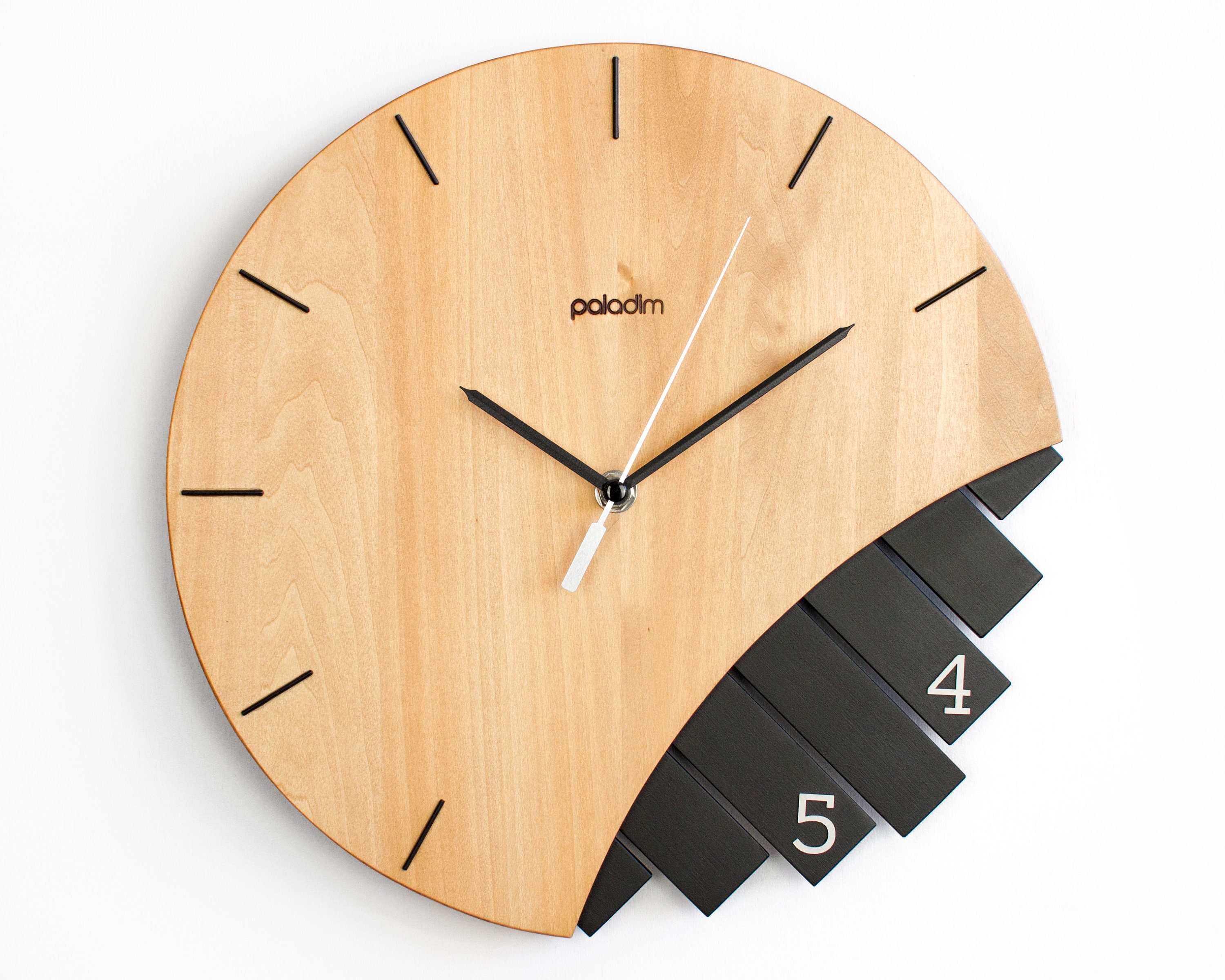This indoor photograph captures a unique wooden clock set against a plain white background, giving it a floating appearance. The clock, made from light-colored wood with horizontal lines, features minimalist hour markers with black slashes for most hours. However, the 3, 4, 5, and 6 positions display something different: at the bottom-right quadrant, the wood is cut away to reveal seven protruding black rectangular pieces. Two of these, corresponding to the 4 and 5 positions, feature white numerals. Beneath the 12 o'clock position, the manufacturer’s name, "paladin," is written in lowercase letters. The clock's hands are slender, with black for the hour and minute hands, and white for the second hand.